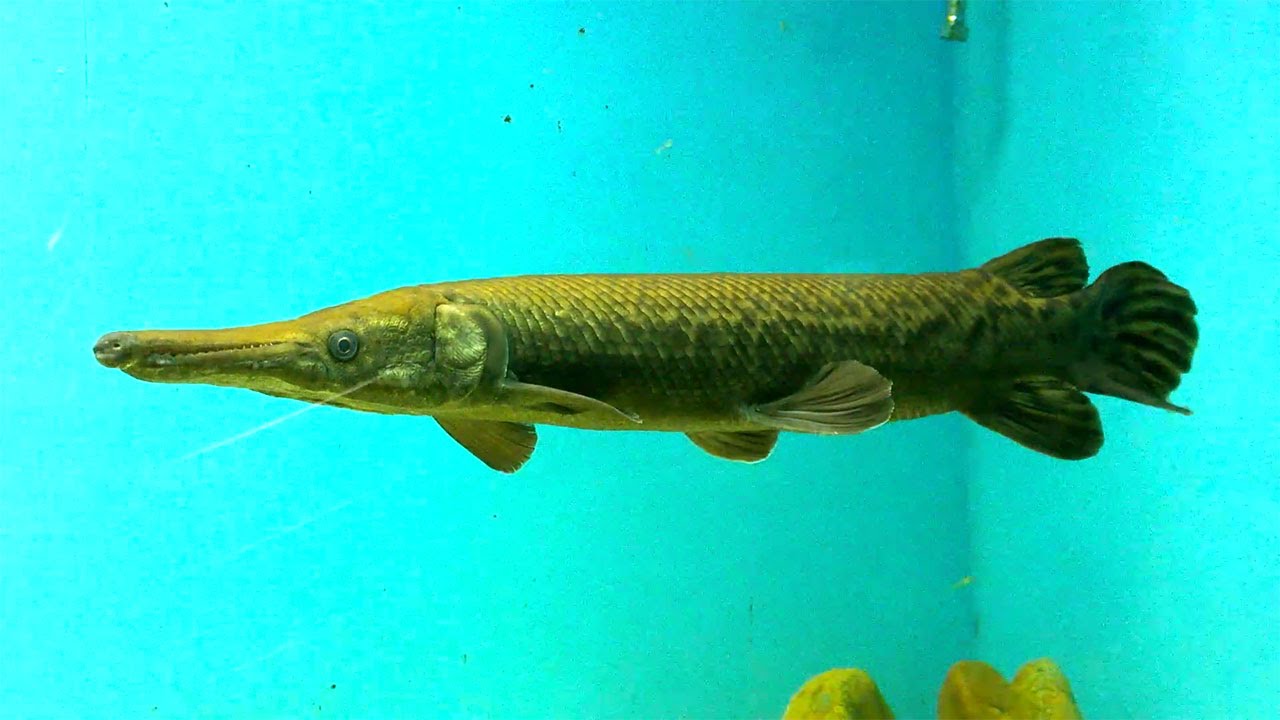This photograph captures a detailed side profile of a long, thin green fish with an almost cylindrical body inside an aquarium. The fish showcases an array of green shades; its body primarily light green adorned with darker green spots. Starting from its elongated, slightly open mouth displaying subtle teeth, to its distinctive black, round eye, the fish presents a striking profile. The head of the fish is on the left side and appears in an olive green hue, while the body transitions into vertical scales of the same color, gradually leading to the tail on the right. The fish has a complex fin arrangement—two pairs of fins positioned along its body and two additional fins right before the tail, which is accompanied by a fin at the top and bottom. 

The background features contrasting blue walls of the aquarium, providing a vibrant backdrop. On the left side, the blue color is lighter, gradually darkening towards the right, suggesting the corner of the aquarium. In the lower right corner, part of a yellow object, possibly coral or a decoration, protrudes into the frame, while the upper right corner contains a small green element. Overall, the photograph is a captivating snapshot focusing heavily on the green fish set against the bright blue aquatic environment.